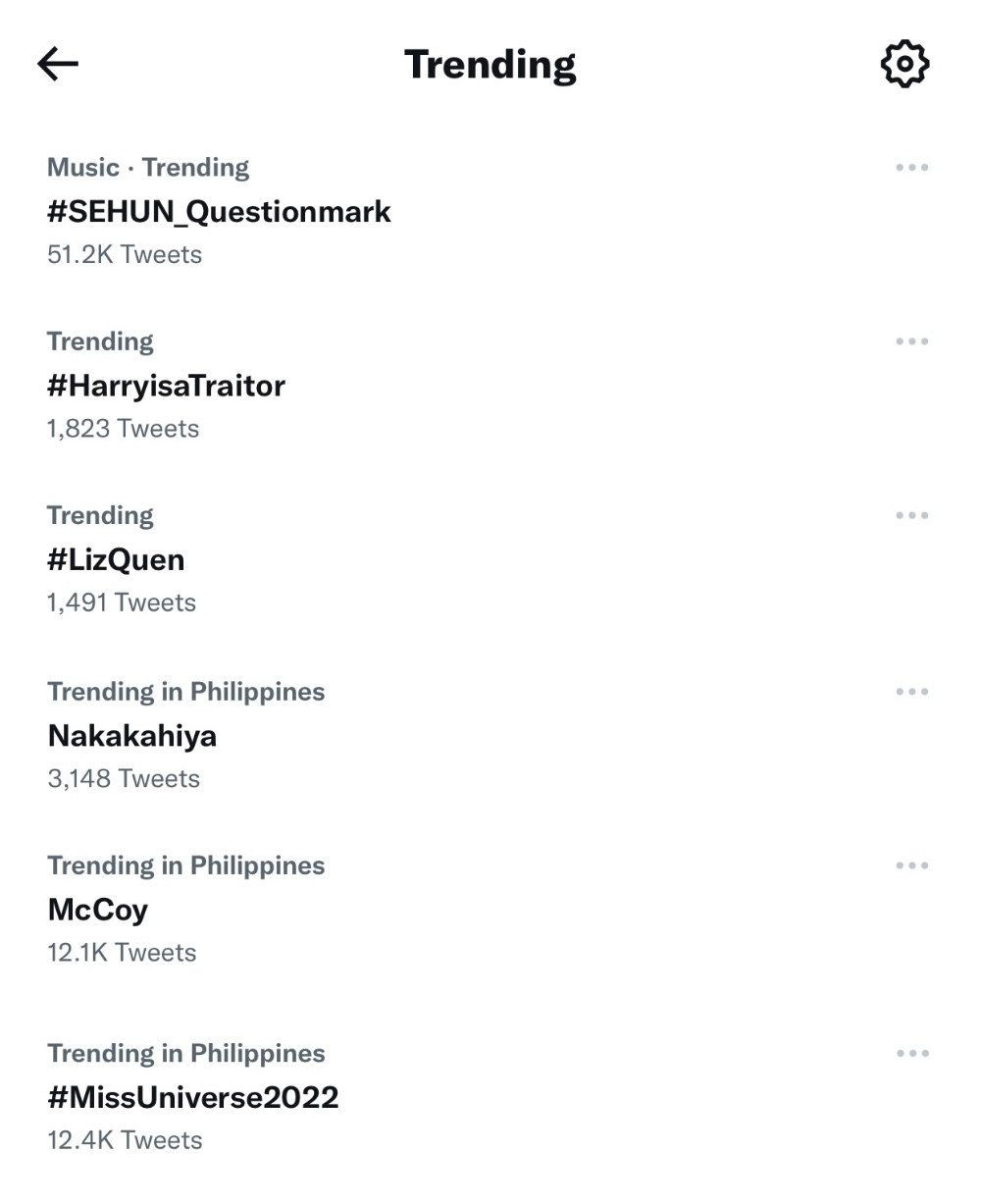Here is a cleaned-up and detailed descriptive caption for the image:

---

The image depicts a section of a website displaying trending topics. At the top of the section, the title "Trending" is prominently featured in bold black letters. To the right of the title is a settings icon, while an arrow pointing left is positioned on the left side.

The first trending topic listed is "Trending in Music," marked by the hashtag "she_hun?" and noted to have 5.2K tweets. To the right of this item are three vertical dots, suggesting additional options.

Below it, another trending topic is "#HarryIsATraitor," with 1,823 tweets, accompanied by three horizontal bars and three vertical dots on the right side. Following this is "#LizQuinn," with 1,491 tweets, and the three dots are likewise present to the right.

Further down, trending in the Philippines, is a topic with 3,148 tweets, also followed by the three dots on the right side. Next is "McCoy," trending in the Philippines with 12.1K tweets, once again featuring the three dots to the right.

Finally, another trend from the Philippines is "Miss Universe 2022," boasting 12.4K tweets, and similarly accompanied by the three dots on the right.

The entire list is presented in simple black text against a stark white background, indicating the trending hashtags and their tweet counts without any additional visuals.

---

This detailed caption captures the visual elements and context of the website screenshot comprehensively.